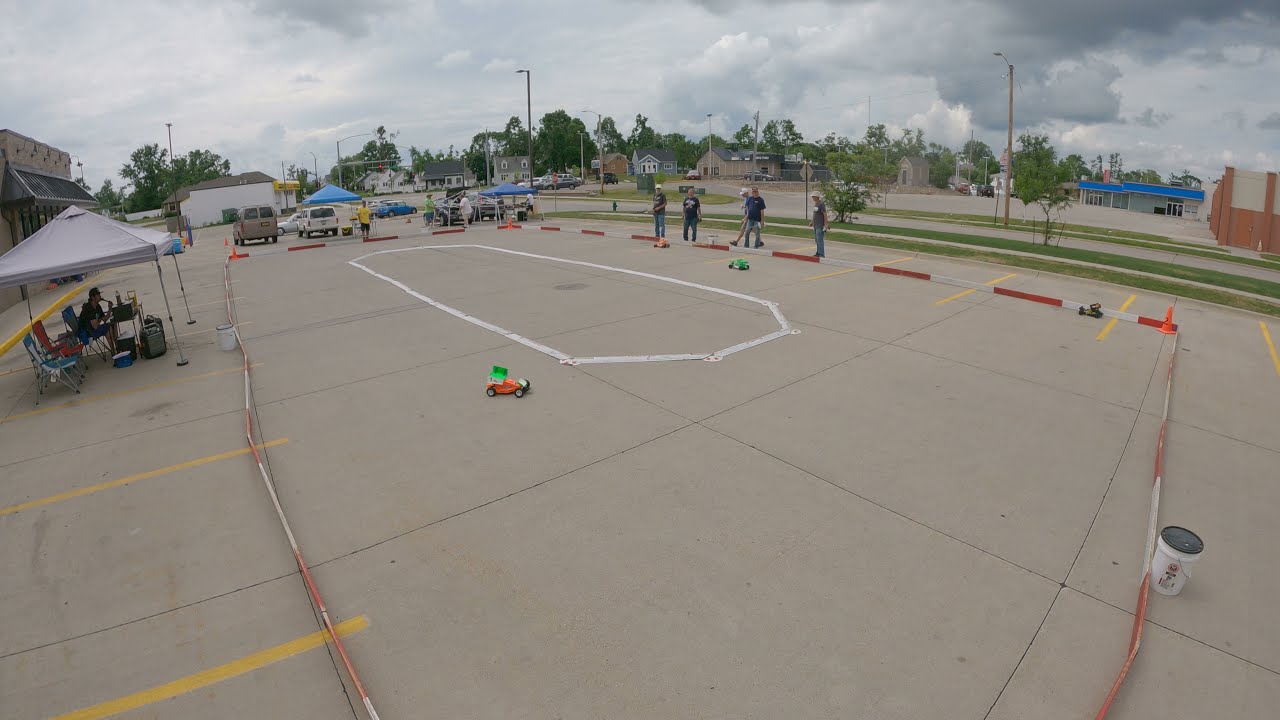In the photograph, we see an outdoor scene on a large, concrete lot surrounded by lush green trees. The sky above is filled with numerous clouds, creating a somewhat overcast day. Central to the scene is a makeshift racetrack, delineated by a white-bordered oval made from masking tape and cardboard. Various remote control cars, including green and orange ones, are zooming around the track, driven by people holding remotes. 

The area is bustling with activity; several blue canopies are set up, presumably for vendors selling items. A group of camping chairs is positioned near a canopy on the far left, where a person is seated amidst luggage bags. To ensure safety and organization, the track area is cordoned off with red-and-white striped barriers and traffic cones. 

In the background, a main road is visible, flanked by another parking lot with multiple parked cars, highlighting the location's access and busy nature. The photograph captures the lively atmosphere of a community enjoying a day of outdoor fun with remote control car races.